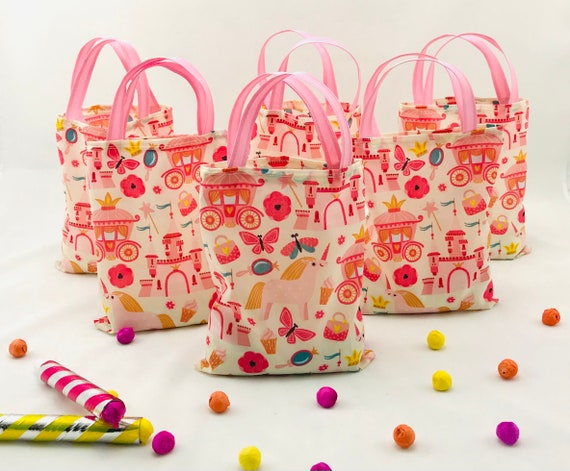The photograph is a delightful scene set against a white background, featuring a white table adorned with six festive party bags. Each bag has sturdy pink handles that stand up straight and is decorated with vibrant, princess-themed illustrations. These illustrations include whimsical elements like a royal carriage, butterflies, unicorns, flowers, ice cream, handbags, and a castle, all in shades of pinks, blues, and oranges. In front of the bags, colorful candies or perhaps small cereal pieces in hues of orange, yellow, and purple are scattered on the table, adding to the playful atmosphere. Additionally, on the left side of the table, there are two coiled containers with spiral colored designs in red and yellow, possibly serving as party favors or noise makers. This charming arrangement is lit by an overhead light, enhancing the vivid colors and joyful feel of the setting.